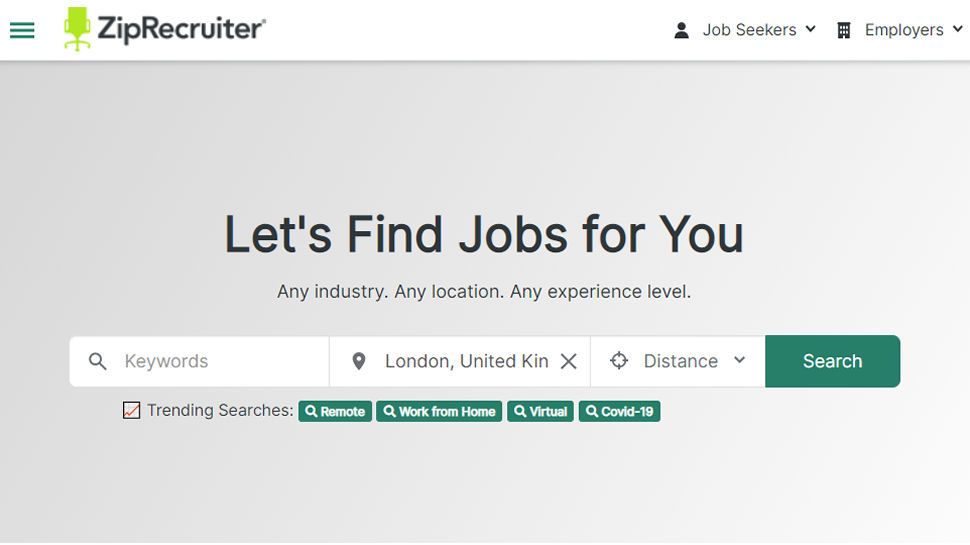This vertical image, captured from a smartphone or computer screen, features the interface of the ZipRecruiter application with a predominantly gray background and a white top section mimicking the computer's screen color. Situated at the top left are three green vertical lines and a lime green chair icon, adjacent to the bold, black text "ZipRecruiter." To the right, there's a small person icon followed by the options "Job Seekers" and "Employers," with arrows indicating additional selections.

Beneath these elements lies a large gray horizontal rectangle featuring the prominent, bold black headline, "Let's Find Jobs For You." Below in smaller, less bold font are the phrases "Any industry, any location, any experience level." A white rectangular input box follows, labeled with "Keywords, London, United Kingdom, Distance," and includes a search bar for input.

Further down, green boxes with white text highlight "Trending Searches" such as "Remote," "Work From Home," "Virtual," and "COVID-19." To the left of "Trending Searches" is a small black square, marked by an orange checkmark, indicating it has been clicked.